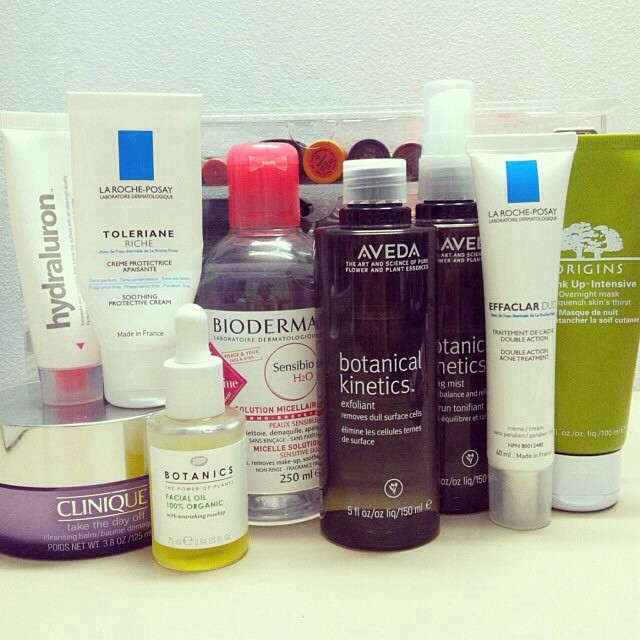A close-up of a white countertop teeming with an array of assorted beauty products. From left to right, the products are meticulously arranged, showcasing various recognizable brands. Notable among them, a transparent jar with a gold-colored lid holds a Clinique product, and perched atop it is a tube of Hydraluron. Adjacent to these, a white squeeze bottle from La Roche-Posay stands prominently. A clear dropper bottle filled with yellow-hued oil, labeled "Botanics Face Oil 100% Organic," is also visible. Additionally, there is a clear plastic bottle with a red cap labeled Bioderma. The assortment continues with products from Aveda and Origins, including a distinctive lime green squeeze bottle from Origins. In the background, lipsticks and chapsticks are neatly arranged against the wall, completing the organized yet abundant display of beauty essentials.